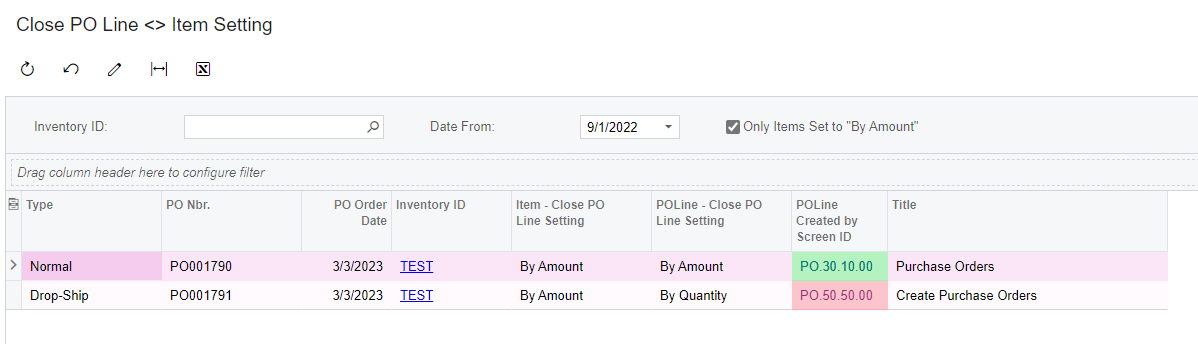The image depicts a user interface for managing purchase orders (PO). At the top, there's a header with the text "Close PO Line" and an icon with two triangles facing each other. Below that, there is an "Item Setting" section which includes an inventory ID field accompanied by a search bar. It shows a date set to "9-1-2022" and features a dropdown menu for more options. A checkbox is marked for "Only items set to by amount."

The interface also has an instruction that reads "Drag column heading to configure filter," followed by a list of column headers: "Type," "PO Number," "PO Order Date," "Inventory Item Closed," "PO Line Setting," "PO Line Closed," "PO Line Setting," "PO Line Created By," "Screen ID," and "Title."

Further down, there are data entries highlighted in colors for different status indicators. In pink, "Normal" is displayed next to "PO001790332023," labeled as "Test by Amount PO.30.10.00." Below that, another entry is marked as "Drop Ship PO001791332023," labeled as "Test by Amount by Quality PO.50.50.00," also in pink. Lastly, a green highlighted status indicating "Purchase Orders" is present, and at the bottom, there's a button labeled "Create Purchase Orders."